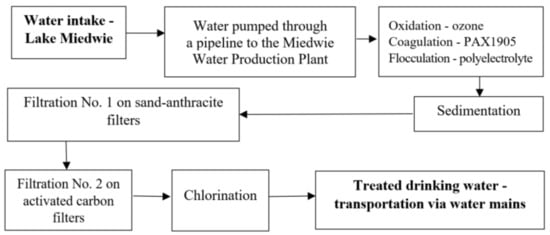This flowchart, set against a solid white background, details the water treatment process for Lake Miedwie. The sequence begins with a bolded rectangle in the upper left corner reading "Water intake - Lake Miedwie". A rightward arrow leads to a box stating "Water pumped through a pipeline to the Miedwie Water Production Plant." Another arrow points to a rectangle listing the stages "Oxidation - ozone, Coagulation - PAX-1905, Flocculation - polyelectrolyte." Following the treatment stages, a down arrow leads to "Sedimentation." From there, a long left-pointing arrow directs to "Filtration number 1 on sand-anthracite filters." Another down arrow leads to "Filtration number 2 on activated carbon filters" located in the lower left corner. A rightward arrow moves to "Chlorination," followed by another arrow leading to a final bolded rectangle in the lower right corner that reads "Treated drinking water - transportation via water mains."